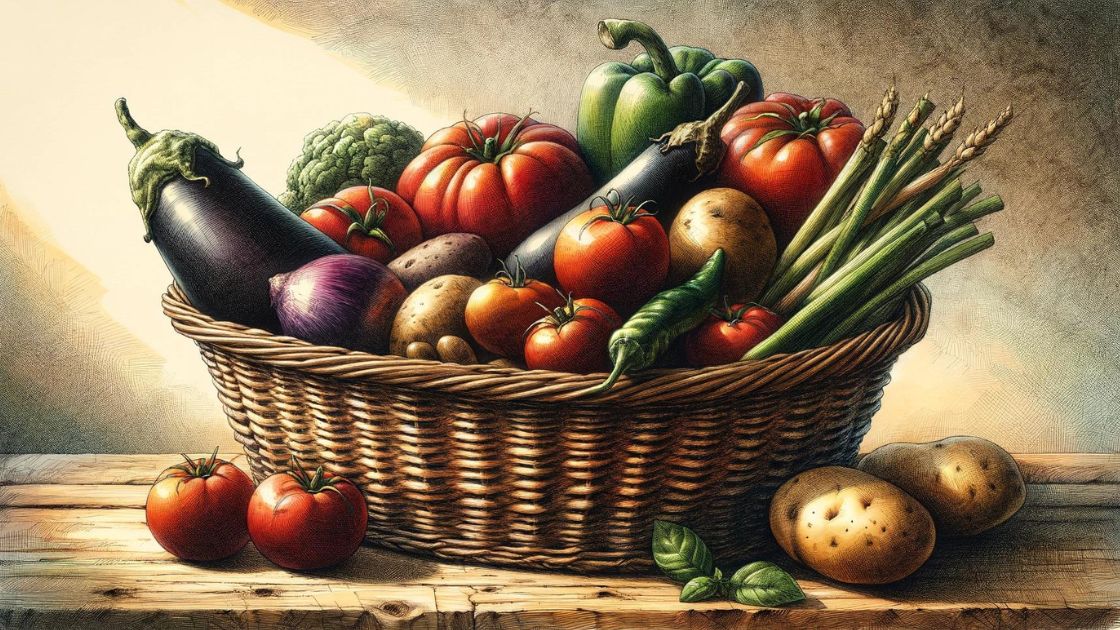This artistic rendering depicts a beautifully detailed basket of vegetables, emphasizing their vibrant colors and fresh appearance. The oval, dark brown wicker basket is set on a rough wooden table. Outside the basket, to the left, are two perfectly round red tomatoes with stems intact. On the right, there are two light tan potatoes with small indents. Adjacent to the potatoes is a sprig of mint with three small leaves.

Inside the basket, a diverse array of produce is meticulously arranged. Prominently displayed are multiple red tomatoes, a bunch of asparagus, a green pepper, a purple onion, an eggplant to the left, another eggplant in the center diagonally, a head of broccoli, and several more potatoes. The background features a textured wall in varying shades of brown and tan, resembling old plaster, lending a rustic charm to the scene. The overall composition is carefully crafted, making the vegetables appear freshly picked, ready to be turned into a delightful meal.